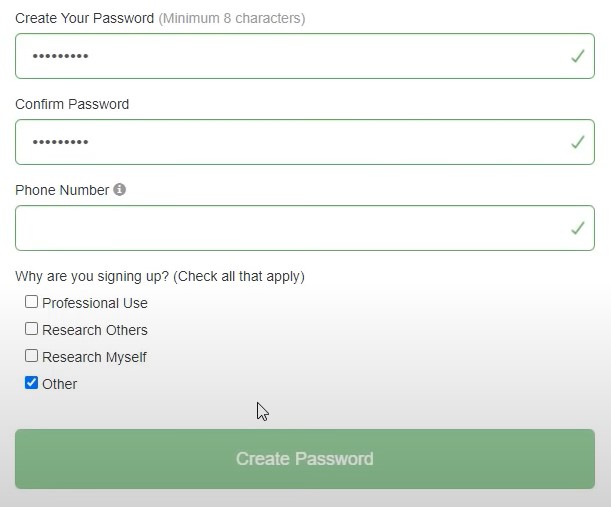The image is a detailed screenshot of a "Create Your Password" page, set against a white background. At the top, "Create Your Password" is prominently displayed in black text, followed by the instruction "(minimum 8 characters)" in grey text. Below this, there's a green-outlined password input box containing nine obscured characters represented by dots, indicating a minimum of nine characters have been entered. On the right side of the password box is a green checkmark, signifying that the password meets the requirements.

Underneath, "Confirm Password" is also written in black text, followed by an identical nine-dot password box and another green checkmark, confirming that both entries match. Below this, there's a prompt for a "Phone Number" accompanied by an information icon. This field is similarly enclosed in a green box with a green checkmark to the right, implying the required phone number has been correctly entered.

Further down, the form asks, "Why are you signing up?" with the instruction "check all that apply" in parentheses. This section includes several checkboxes: "Professional Use," "Research Others," and "Research Myself" are all unchecked, while "Other" is checked, indicated by a blue box with a white checkmark.

A cursor is visible hovering slightly above the center of a green "Create Password" button at the bottom of the form. The text on the button is somewhat grayed out, suggesting that additional information—presumably the phone number—needs to be completed before the button becomes fully active and the account creation process can be finalized.